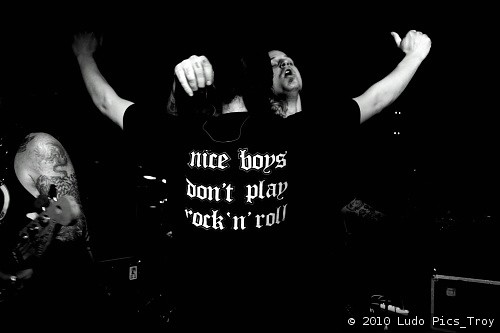In this black and white photograph, three individuals are captured in an indoor setting that exudes an ambiance akin to a concert. The focal point of the image is a person in the center, wearing a black short-sleeved T-shirt adorned with the bold white text, "Nice boys don't play rock and roll" arranged in three rows. This person is standing with both arms raised, giving a thumbs-up gesture. Directly in front of this central figure, a man is caught in a moment of ecstasy, his head thrown back and his hand reaching over the shoulder of the person in the black T-shirt as if embracing him. To the left, partially visible, is another individual with a dragon tattoo adorning their exposed arm; this person holds an electric guitar, hinting at a musical performance setting. The background fades into near-complete darkness, obscuring additional details and creating a heavily shaded atmosphere. A caption in the bottom right corner reads, "Copyright 2010 Ludo Pics Troy," solidifying the professional nature of this captivating and celebratory moment.